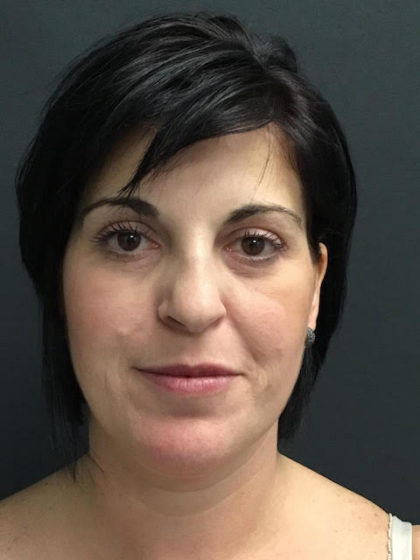This image is a close-up portrait of a woman in her mid-to-late 30s or 40s with short, braided black hair that blends into the mildly sheened grayish-black background. She has a fair complexion and is wearing minimal makeup, with visible mascara and possibly some lip color. Her expressive dark brown eyes are wide open, looking directly at the camera. She has a high forehead and a longer nose. The lighting accentuates her left shoulder, where a white strap of her tank top can be seen. An earring adorns her ear, adding a subtle touch of elegance. The woman's closed-mouth expression, featuring a mild smirk, gives an impression of sadness or contemplation. Overall, her face is the focal point, with her calm yet slightly melancholic demeanor captured poignantly in this head shot.